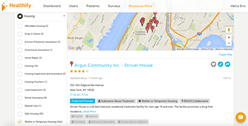At the top right corner of the image, there is a rectangular section of a map showing the bottom portion of a geographic area. Scattered across the middle of the map are several red pins, two of which—the one in the center and another to the left—feature a black dot at their centers. 

On the far left side of the map, an expanded menu is visible. The menu starts with a light gray header featuring a black icon on the left and some black text next to it. To the right of the text, there's a down-pointing arrow, indicating a dropdown menu that is currently open. Below the header, several items in black text are listed in a column, each next to a square checkbox with a gray border. The bottom-most checkbox is checked off with an orange check mark.

In the top left corner of the page, there is an orange icon resembling an upside-down triangle. To the right of this icon, a logo, possibly reading "Healthify," is partially visible but hard to decipher. 

Further to the right, there are five menu options in black text, with the fifth option highlighted in orange, possibly labeled "Restaurant Menu." Continuing to the right side of the highlighted option is an additional segment of black text.

Beneath the map, a red pin is shown alongside a line of light blue clickable text that includes the words "community" and the abbreviation "ink," separated by a dash. Directly below this text are four yellow stars.